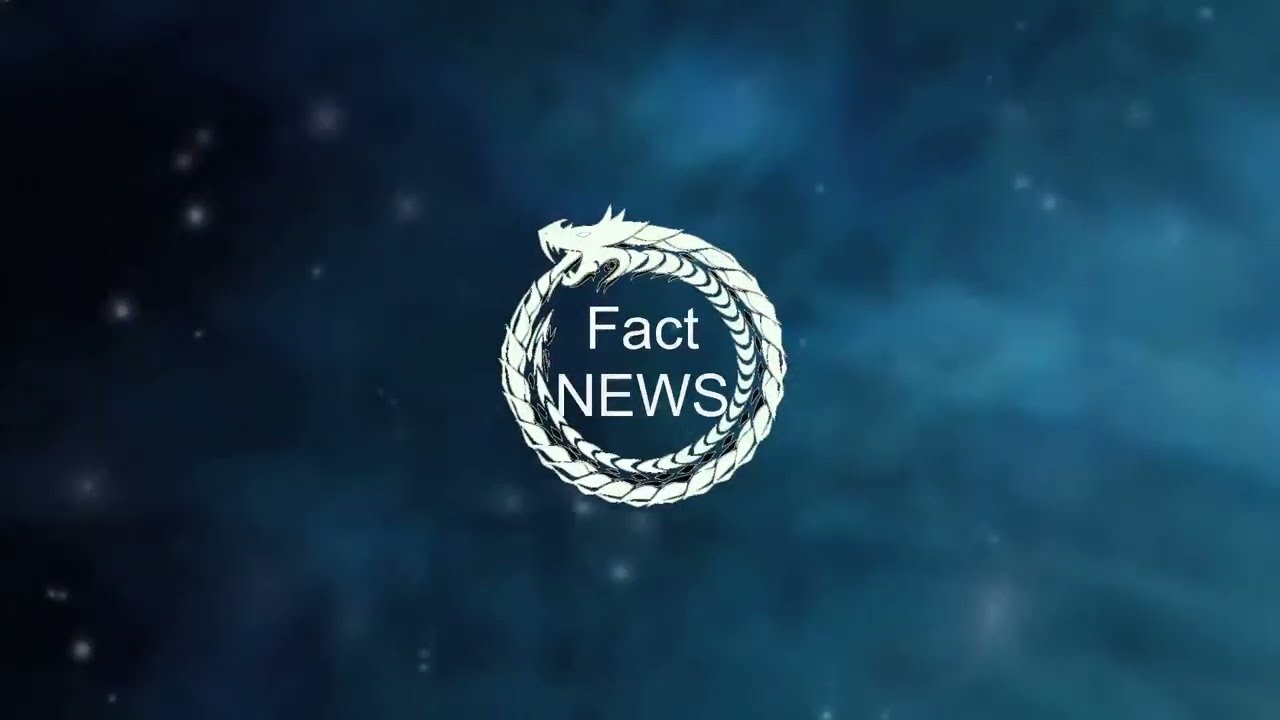The image features a mottled green background with areas of dark blue on the left and lighter blue with some white and blurry steam on the right. In the center is a minimalist, white symbol of a dragon eating its own tail, an ouroboros, positioned with its head at approximately 11 o'clock. The dragon appears as a thickening rope that nests within itself, forming a continuous circle. In the inner space of the dragon's encirclement, there is white sans serif text with "Fact" capitalized at the top and "NEWS" in all caps at the bottom. The colors and simplistic design elements create a stark contrast that emphasizes the central symbol and text.